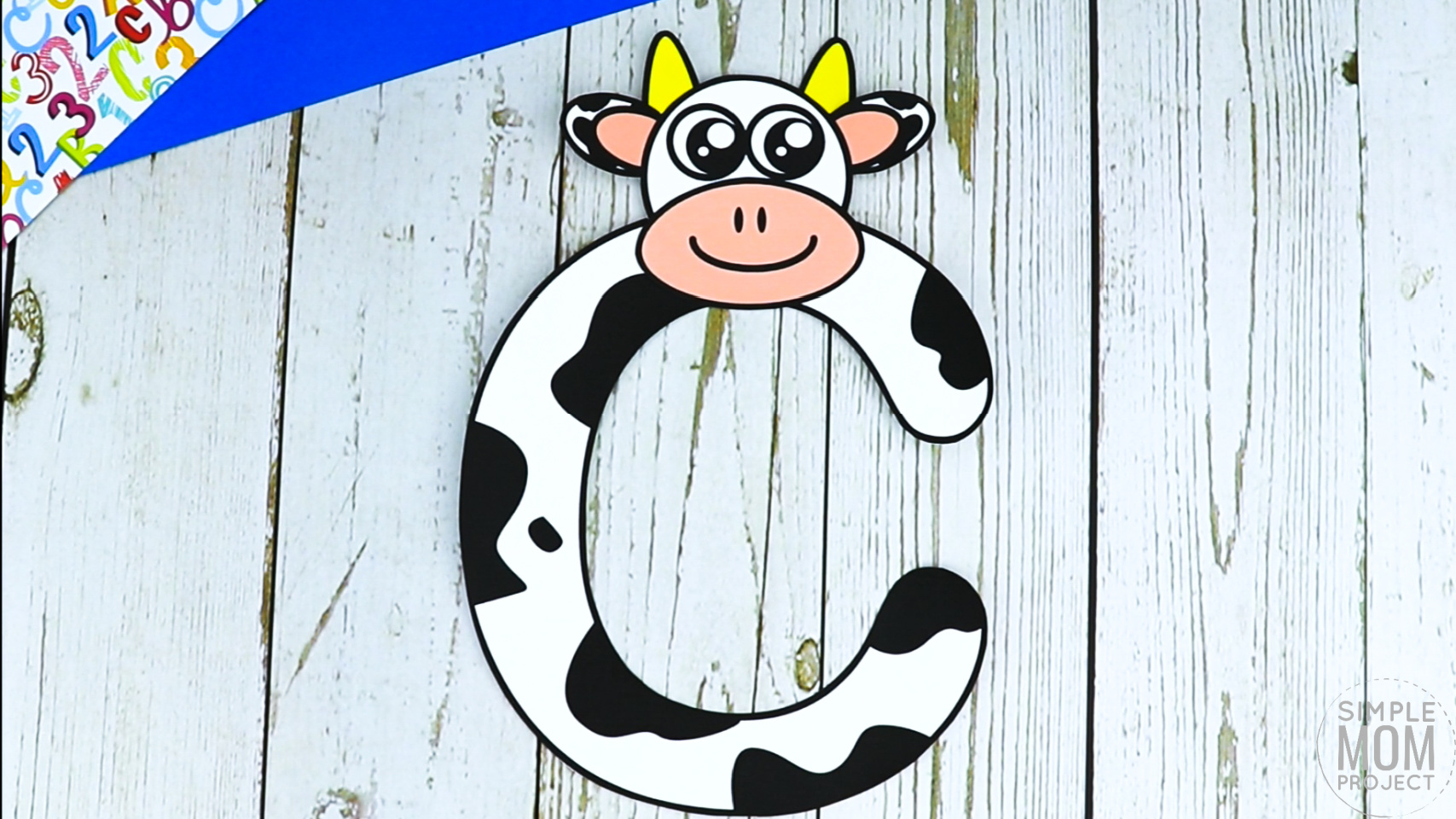The image depicts a playful illustration where the letter "C" is transformed into a cow. The body of the letter is white with black splotchy patches, mimicking a cow's hide, with the head of a cartoon cow perched on top. The cow's head features large, expressive eyes, a smiling face, pink and black ears, and yellow horns. The inner parts of its ears are a pinkish-beige color matching its snout. This whimsical "C" rests against a background resembling a light-colored or distressed wooden fence, potentially with streaks of paint. In the upper left corner, there is a colorful triangle adorned with various letters, predominantly "C," and numbers such as "2" and "3." Adjacent to it is a smaller plain blue triangle. At the bottom of the image, a logo within a circle reads "Simple Mom Project."